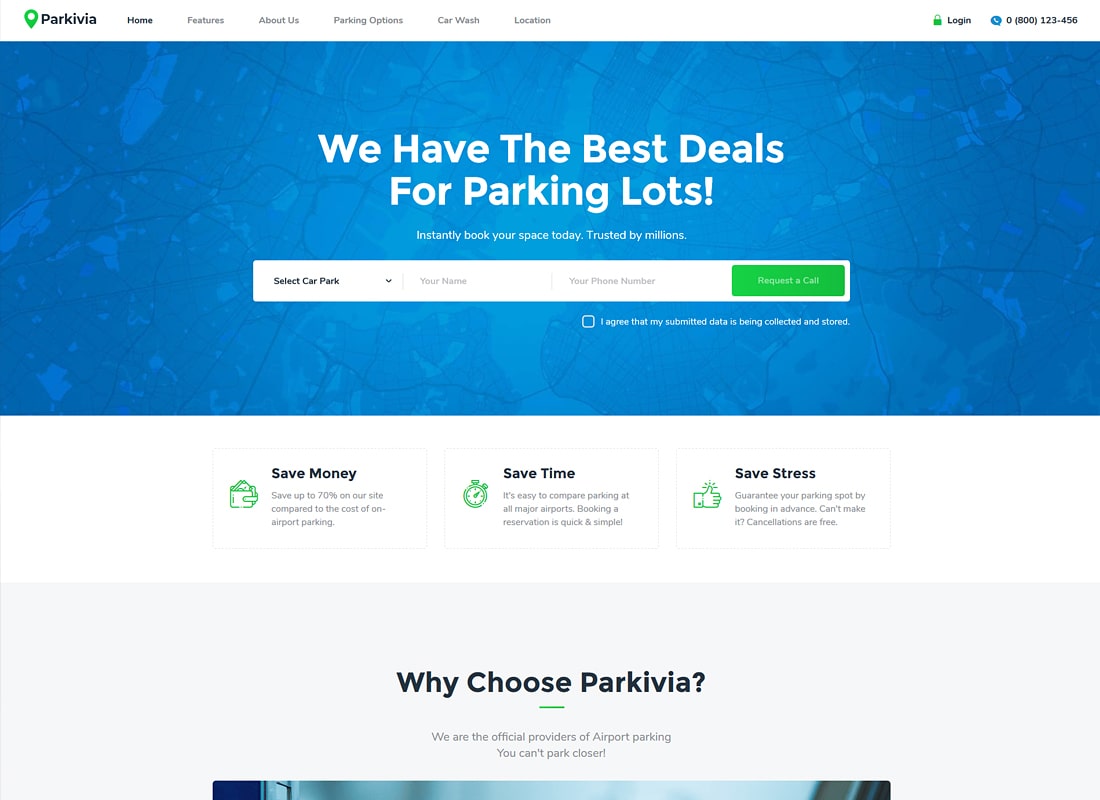This is a highly detailed screenshot of a website mock-up, likely a template available for purchase. The design features a common layout with various elements aimed at a parking services website for a company named "Parkivia," located in Texas.

In the top left corner, there is a green map pointer icon highlighting Parkivia's location. To the right, a navigation menu is displayed with "Home" pre-selected, followed by links to "Features," "About Us," "Parking Options," "Car Wash," and "Location." Further to the right, there’s a green lock icon adjacent to a "Login" link, a telephone icon, a text bubble icon, and a customer support phone number: 800-123-456.

Beneath the header, there's a prominent hero image that appears to resemble faux stone or marble, tinted in various shades of blue with vein-like patterns. Superimposed on this background is the headline, "We have the best deals for parking lots," in white text, with a subheading beneath that reads, "Instantly book your space today, trusted by millions."

The interactive section below the heading includes a white rectangular dropdown menu labeled "Select Car Park," followed by input fields for "Your Name" and "Your Phone Number." A green "Request a Call" button is positioned below these fields. Additionally, there is an unchecked white checkbox labeled, "I agree that my submitted data is being collected and stored."

Below this form, the website features a section with three icons: a wallet (save money), a stopwatch (save time), and a thumbs up (save stress), each accompanied by brief descriptions. Further down, a statement in white text reads, "Park here, we're the only official provider of airport parking. You can't park closer."

The footer of the screenshot appears to have an incomplete JPEG cut off at the bottom, adding to the template’s unfinished appearance.